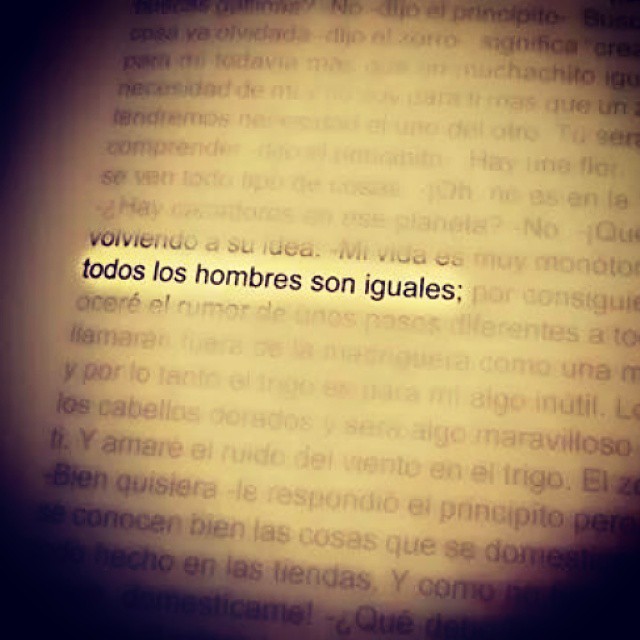The image depicts a page taken from a book or magazine, featuring a predominantly yellowish-brown background with black lettering. The page is mostly blurred, creating a sense of shadowing and a dark backdrop. This blurring effect accentuates a central focal point where a single line of text is clearly legible: "Todos los hombres son iguales," which translates to "All men are equal." This highlighted line appears within a circular area, as if illuminated by a spotlight, drawing intense focus to the message. The background remains obscure, with only the focused line standing out amidst the blurred text, emphasizing the idea of equality conveyed by the clear Spanish phrase. The overall presentation of the image is intriguing, making the highlighted message the central point of attention.